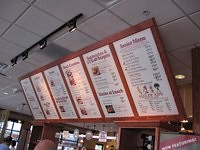In this photograph, an industrial-style restaurant interior is depicted. The ceiling is composed of white acoustic tiles framed by metal strips. A prominent menu board is mounted at an angle, directing patrons' attention downward. It features six individual panels, each separated by narrow brownish dividers that resemble wood. The border of the sign is similarly brown. Though the image is small and unclear, the menu panels appear to have headings at the top, likely indicating different categories such as drinks, sandwiches, salads, side dishes, and desserts. Some panels include images, presumably showcasing the food items available. Despite the blurred details, the sign seems to provide descriptions and prices for each item. A window in the distance adds depth to the scene, although the specifics of the view are indiscernible.